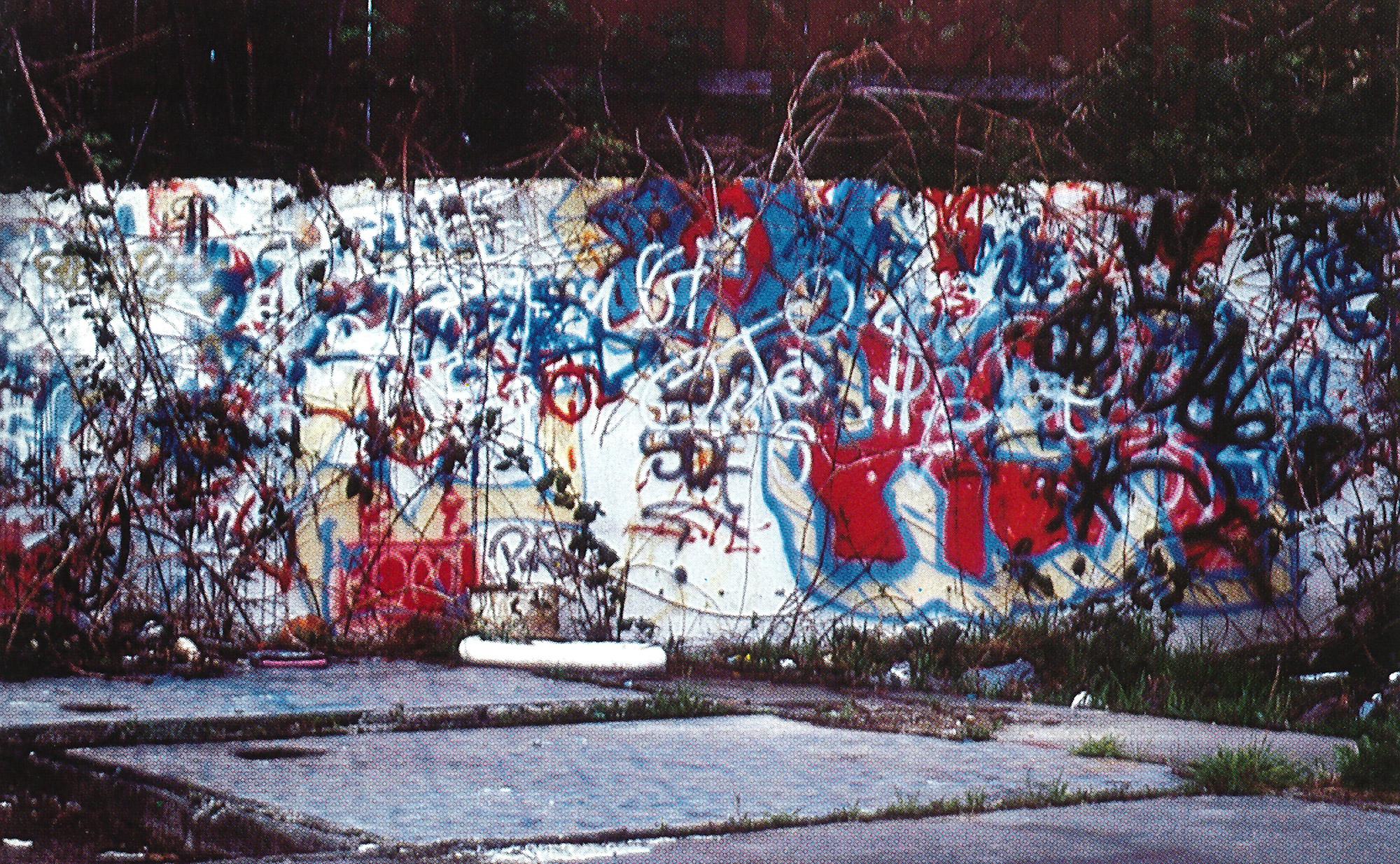The image depicts a wall covered in elaborate and colorful graffiti that appears inspired by abstract expressionism, reminiscent of Jackson Pollock's style. The wall stretches broadly from right to left and features a diverse palette, predominantly using hues of white, black, red, and blue, with occasional touches of yellow. On the right side of the wall, almost centrally located, is a prominent white dollar sign. Above this, there is a black crown amidst various black scribblings. The surface of the wall is extensively adorned with splashes and layers of paint, resulting in a chaotic yet deliberate composition of jagged lines and symbols.

In the foreground, tall, brown grasses stand out against shorter green grasses, suggesting an outdoor setting, possibly an alley or an exterior wall. This impression is further reinforced by the presence of trees in the background, silhouetted against the night, indicating that the photo was taken after dark. Near the base of the wall, there are three light gray rectangular shapes on what appears to be a cement pathway, possibly wet. Parts of a building with a reddish hue can be seen behind the graffiti-covered wall, further anchoring the scene in an urban environment. The entire scene is dimly lit, likely by some form of street lighting, casting the graffiti in a dramatic glow amidst the darkness.